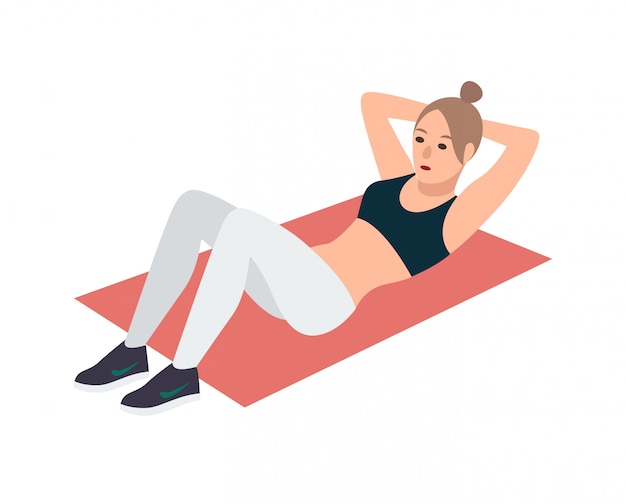This is a computer-generated, cartoon-style image of a woman exercising on a reddish-orange yoga mat. The background is entirely white, drawing full attention to the detailed representation of the woman. She has light brown hair tied in a bun with loose strands forming a U-shape around her forehead. Her complexion is white, and she is doing sit-ups with her hands behind her head and her knees bent at a 45-degree angle. She is wearing a black sports bra and white leggings, matched with black and white Nike sneakers featuring a green swoosh. The woman has red lipstick, a brown nose, and cartoonish black eyes, emphasizing the 2D clip art style of the image.